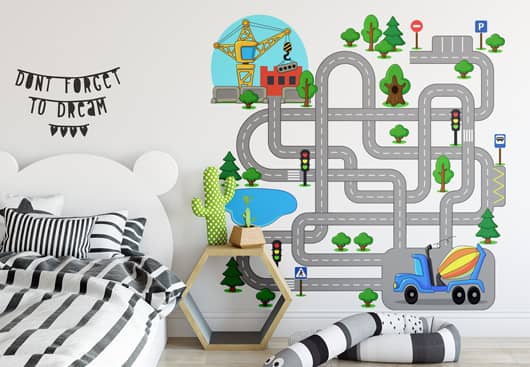This is a staged photo for an advertisement of a child's bedroom, tastefully decorated in a soft gray color palette. The focal point is the white bed with a headboard that resembles Mickey Mouse ears, adorned with black and white, as well as gray-striped pillows and bedding. Above the bed, black lettering on the wall says, "Don't forget to dream," with four heart shapes hanging beneath it. Adjacent to the bed, a wooden bedside table holds a plush cactus and is accompanied by another stuffed cactus beside it. On the wall to the right, there's a unique feature: a wall-mounted maze resembling a child's play mat, complete with roads, trees, traffic signals, a crane at the top, and a dump truck at the bottom. In front of the bed lies a body pillow shaped like a snake, also in gray, black, and white stripes with two eyes. The entire room gives off a cozy, imaginative, and whimsical vibe.